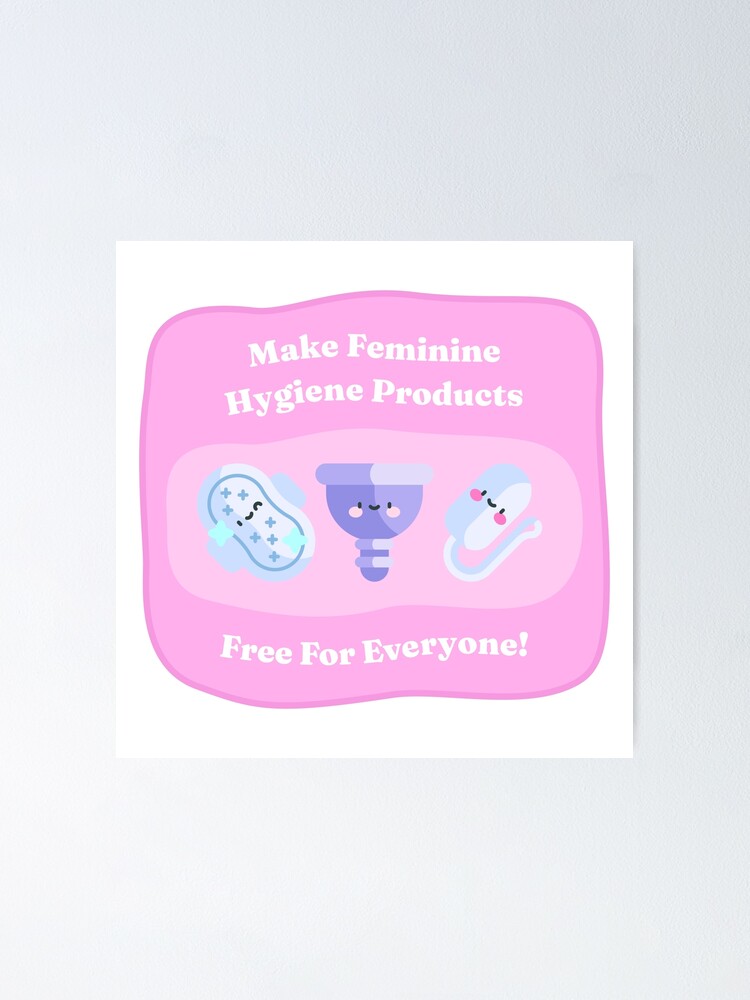The image is an advertisement set against a white square background with a pink border. In the middle of the square, there is a vibrant pink area containing engaging clip art of feminine hygiene products. At the top, bold white letters with all initial capitals proclaim, "Make Feminine Hygiene Products." Below this text, we see three animated characters representing different feminine hygiene products, each with friendly faces. From left to right, there is a white pad featuring small blue X's, a purple menstrual cup with blush on its cheeks, and a white tampon. Beneath these characters, the phrase "Free for Everyone!" is prominently displayed in white capital letters, emphasizing the accessibility of these products. The primary colors in the image are white, pink, purple, and blue, creating a lively and eye-catching theme.